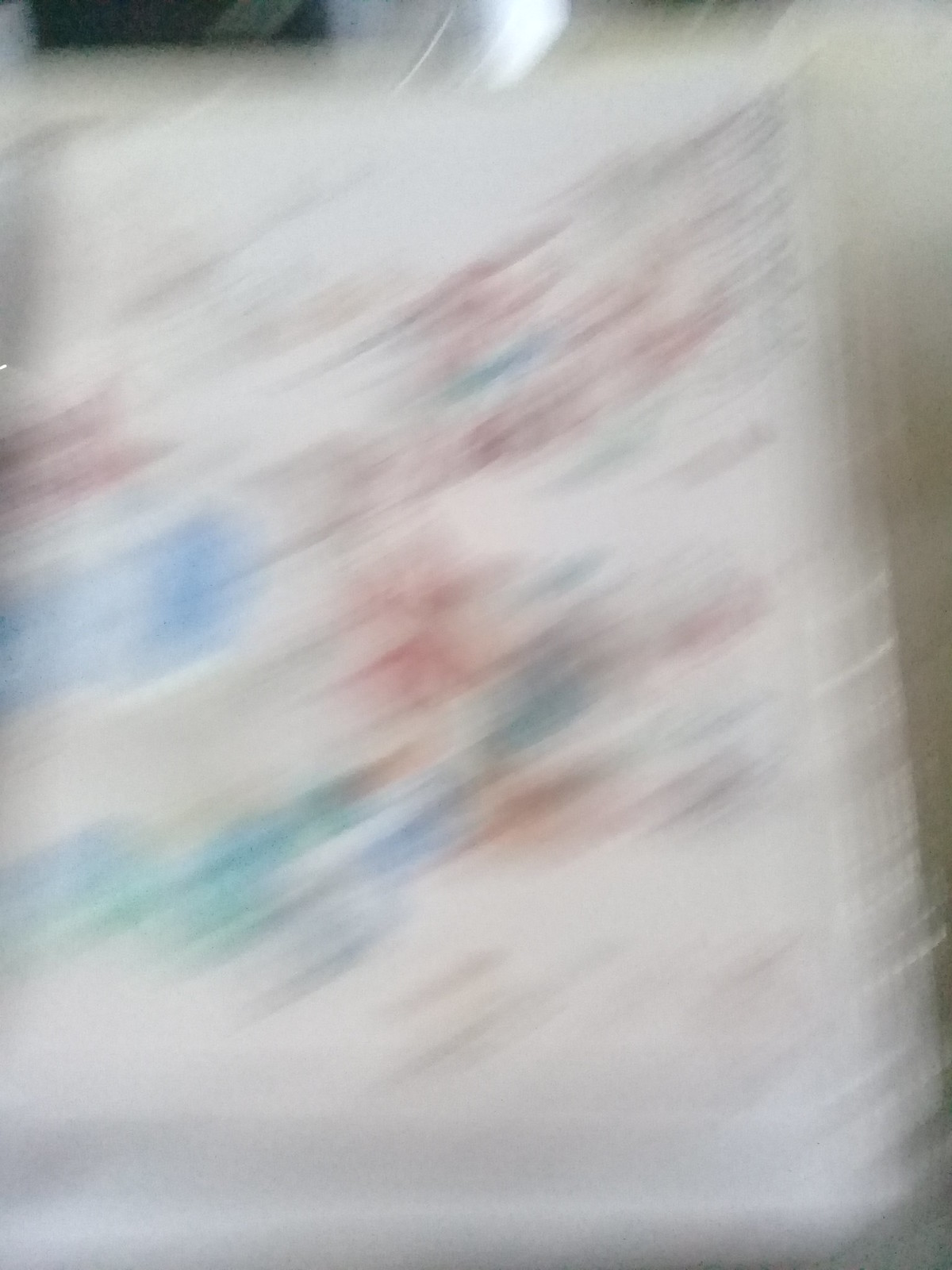The photograph depicts a highly blurred scene, possibly due to the movement of the photographer. The primary focus of the image is a piece of white paper set against a backdrop. On the paper, there are various colors including light blue, pink, dark blue, and purple, all smeared or blurred together in a diagonal pattern from the lower left corner swooping upward towards the upper right corner. The image also features some form of drawing or writing on the paper, but the extreme blurriness makes it impossible to discern any details. Beyond the paper on the left-hand side, there is a long, skinny black rectangle and a small triangular patch of bright white light, providing a stark contrast to the surrounding colors. Overall, the scene appears chaotic and indistinct, with colorful streaks and unclear elements adding to the sense of motion and blur.